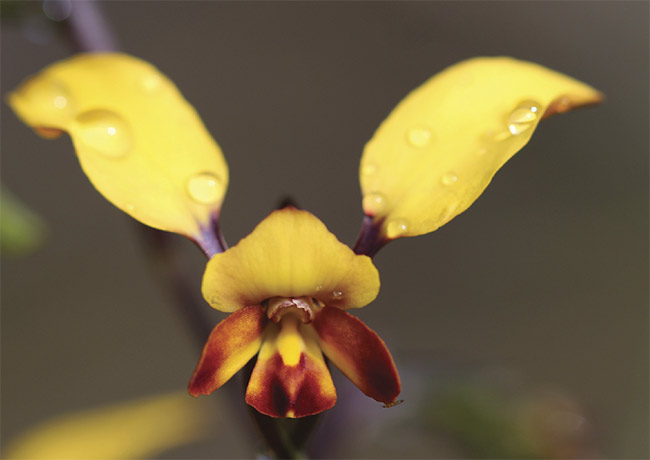This is a close-up photograph of a striking flower, set against a blurred, dark gray background with subtle streaks of yellow and purple. The flower, resembling an orchid, features a total of six petals. Dominating the top of the flower are two longer yellow petals with brown accents at their bases, resembling floppy bunny ears, adorned with clear raindrops and morphing into purple stems. At the center, a prominent yellow petal stands out like a crown, flanked by three maroon petals below, each accented with yellow shadings and spots. The central structure of the flower features yellow elements that evoke an open mouth with a protruding tongue. Dewdrops are visible across the flower, adding a fresh, glistening effect.